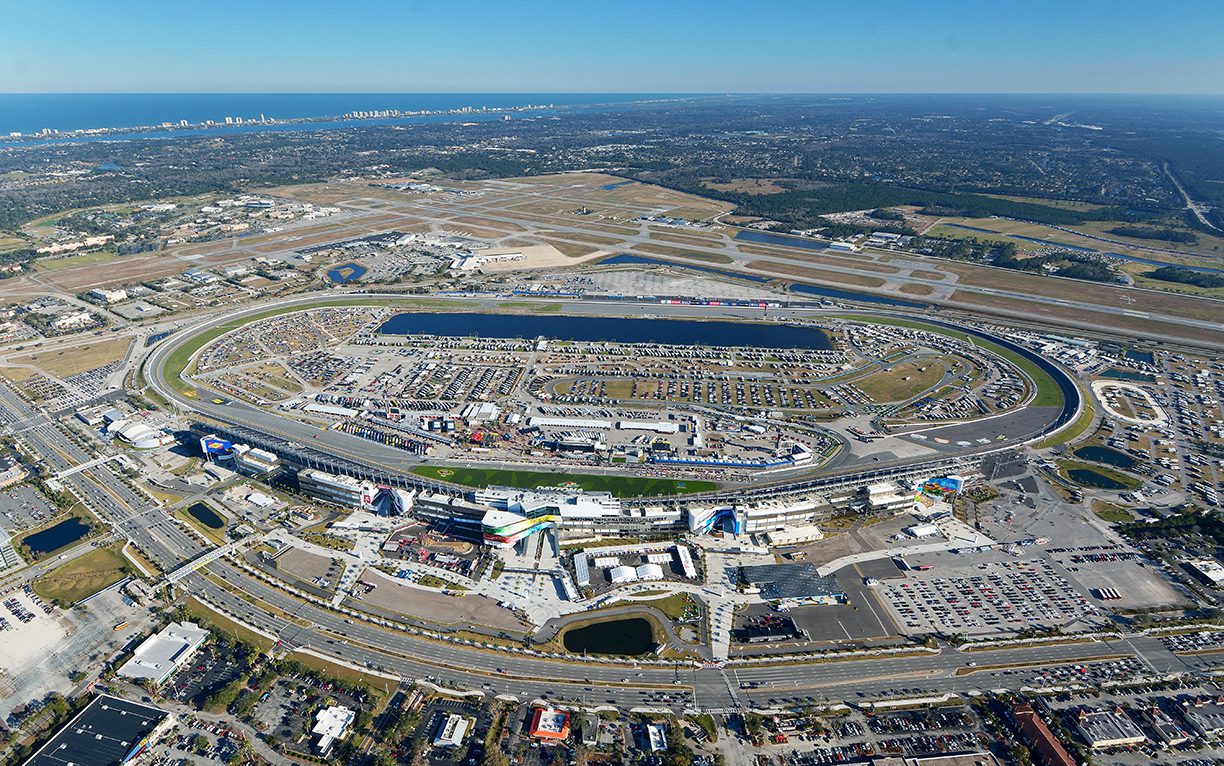This aerial photograph captures an expansive view of a large racetrack complex surrounded by various transportation and commercial areas. Central to the image is the enormous racetrack, teeming with numerous vehicles in its infield, and encircled by a prominent roadway. Several parking lots are scattered around, filled with cars. The racetrack sits amidst a wider infrastructure, with roads intertwining and small cars visible in transit. Adjacent to the racetrack are additional buildings, likely housing businesses or entertainment venues related to the racetrack. To the bottom right and far right, densely packed parking spaces are evident. In the background, a striking expanse of greenery unfolds, leading to what appears to be a distant shoreline, accompanied by a vast body of water, possibly the ocean. Overhead, the image is framed by the clear blue sky, enhancing the breadth and scale of the scene below.